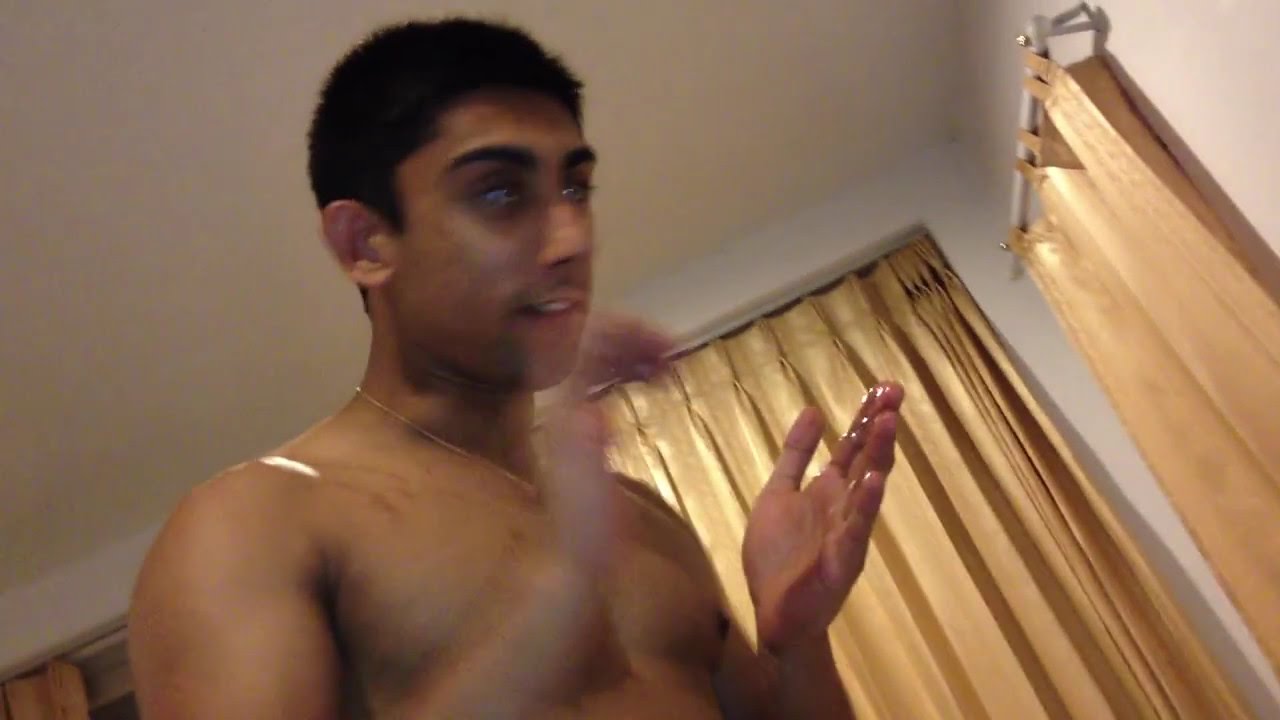The photograph captures a shirtless man, likely in his late twenties or early thirties, standing in the middle of a room. His slightly bronzed skin and short black hair complement his muscular upper body. Adorned with a simple, thin gold chain necklace, he strikes an intriguing pose. His fingers are wet and glistening, suggesting he may have applied some kind of gel. One of his hands appears blurry due to movement, as if he’s clapping or shaking it. His mouth is slightly open, and he looks off to the right, adding a sense of engagement beyond the frame.

The room he occupies features white walls and a white ceiling, with golden curtains adorning the windows and possibly a large sliding glass door behind him. The angle of the photograph is slightly tilted to the left, providing a dynamic and somewhat cinematic perspective. The well-lit room accentuates his wet fingers and offers a detailed glimpse of his expression, which includes a white-toothed smile.